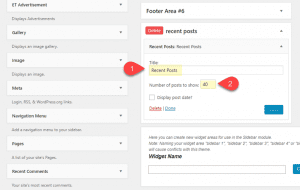This image is a very blurry screenshot featuring a two-column layout with various interface elements. 

On the left column:
- At the top, "ET Advertisement" is displayed in bold black text.
- Below that, there are several white selection fields with gray down arrows on the right side. 
- The second field has "galley" entered, while the third and fourth fields are illegible.
- Further down, a gray section includes the words "Login RSS." The text within the white field in this section is also illegible.
- In the following white field, the word "Pages" is visible at the top. At the bottom, the text reads "Record Credential."

On the right column:
- The top section has a white background with "Footer Area No. 5" and a gray down arrow on the right.
- The next section includes an orange rectangular button with white text, which is unreadable. To its right, "Recent Post" is written with a down arrow.
- Below it, there is black text too small and blurry to discern, except for a section labeled "Title." The title is highlighted in yellow but remains too blurry to read. An orange teardrop shape with a white number "1" is present to the left of this section.
- The next part is labeled "Number of Posts Possibly to Show," with the number "40" shown in a small yellow box. An orange teardrop shape with a white number "2" is to the right.
- Beneath this, there's an unchecked white checkbox accompanied by black text.
- Below this section, an orange "Delete" text appears, followed by "Done" after a pipe symbol. 
- The far right has a rectangular blue button.
- At the very bottom right corner, there's a small, blurry white paragraph.
- Underneath that, "Widget Name" is displayed in bold black. Below it, a white text entry bar is visible with a blue button on its right.

This description aims to provide a detailed and clear representation of the elements and layout within the image.